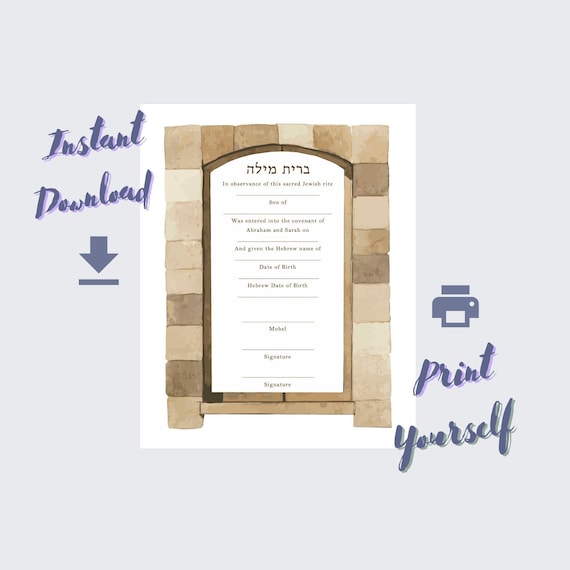The image features a prominently displayed certificate against a purple-gray background. Centered in the image is an invitation or certificate bordered with an array of brown, tan, and off-white blocks, resembling pieces of wood. The inner white border frames the main content which includes writing in Hebrew at the top, likely related to a Jewish ceremony such as a Bar or Bat Mitzvah. The text details spaces for the Hebrew name, date of birth, and other ceremonial specifics. To the left, a "Instant Download" label is accompanied by a downward-facing arrow, both in dark purple. On the right, a printer icon is paired with "Print Yourself," indicating the document is customizable and downloadable. The overall design integrates neutral tones and the font color ranges from blue-gray to purple presented in cursive script, enhancing the elegant aesthetic.